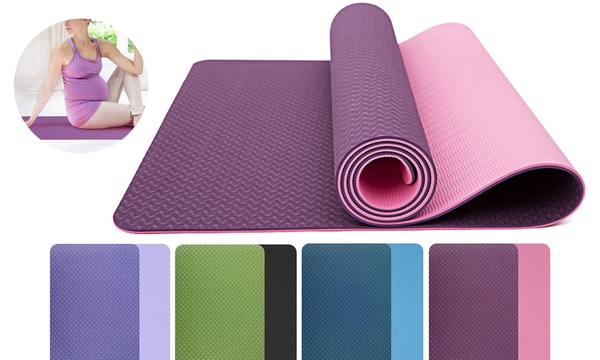This detailed image appears to be an advertisement for yoga mats, showcasing a variety of mats in different colors and configurations. Central to the image is a purple yoga mat that is partially unrolled, revealing its pink underside. Below this main mat are square sample swatches, each depicting a different color combination: a dark steel blue with light blue, an army green with black, and another greenish-blue with cornflower blue. There’s also a close-up of the featured purple and pink mat.

In the upper left of the image, within a circular inset, a woman is shown sitting on the yoga mat. She appears to be pregnant and is wearing light-colored sweatpants and a purple tank top, possibly maternity clothing. Her posture suggests she might be engaging in a yoga pose, with her arms stretched out behind her and her face turned to the side, highlighting the practical use of the yoga mat. The overall arrangement of the mats and the inclusion of the woman creates a cohesive and visually appealing advertisement highlighting the versatility and color options of the yoga mats.